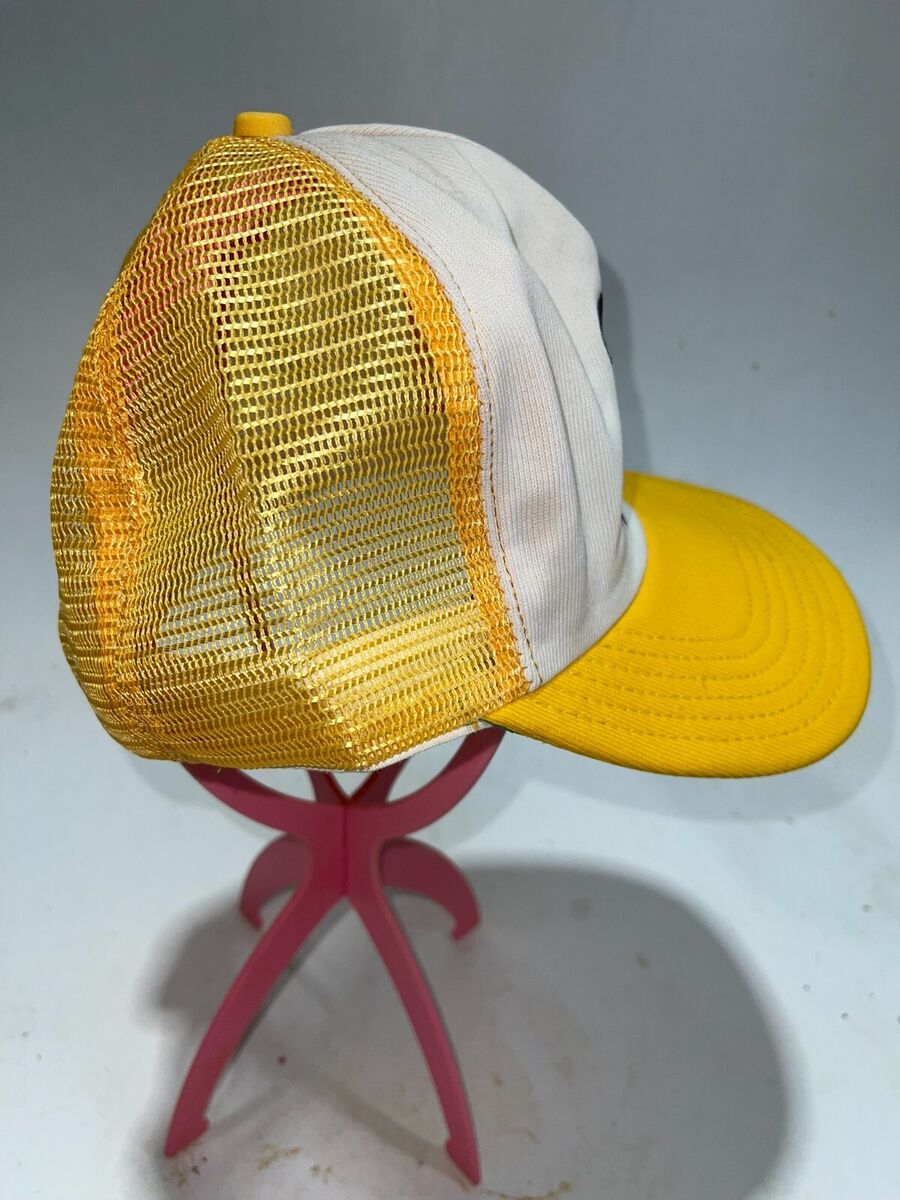The image features a close-up of a baseball cap displayed on an intricate stand. The baseball cap has a bright yellow bill with six visible stitch lines, a yellow mesh back, and a white cloth front. A small yellow knob sits at the pinnacle of the cap where the seams converge. The hat rests atop an unusual stand that mimics the shape of a head. The stand, colored in a vibrant dark pink or purple hue, comprises four thin, widely spaced legs that arch upwards to support the hat. The scene appears to be shot indoors, evidenced by the visible flash shadow on the dirty white table surface below, creating a round shadow under the hat. The detailed structure of both the hat and stand is accentuated by the lighting, highlighting their unique features and contrasting colors.